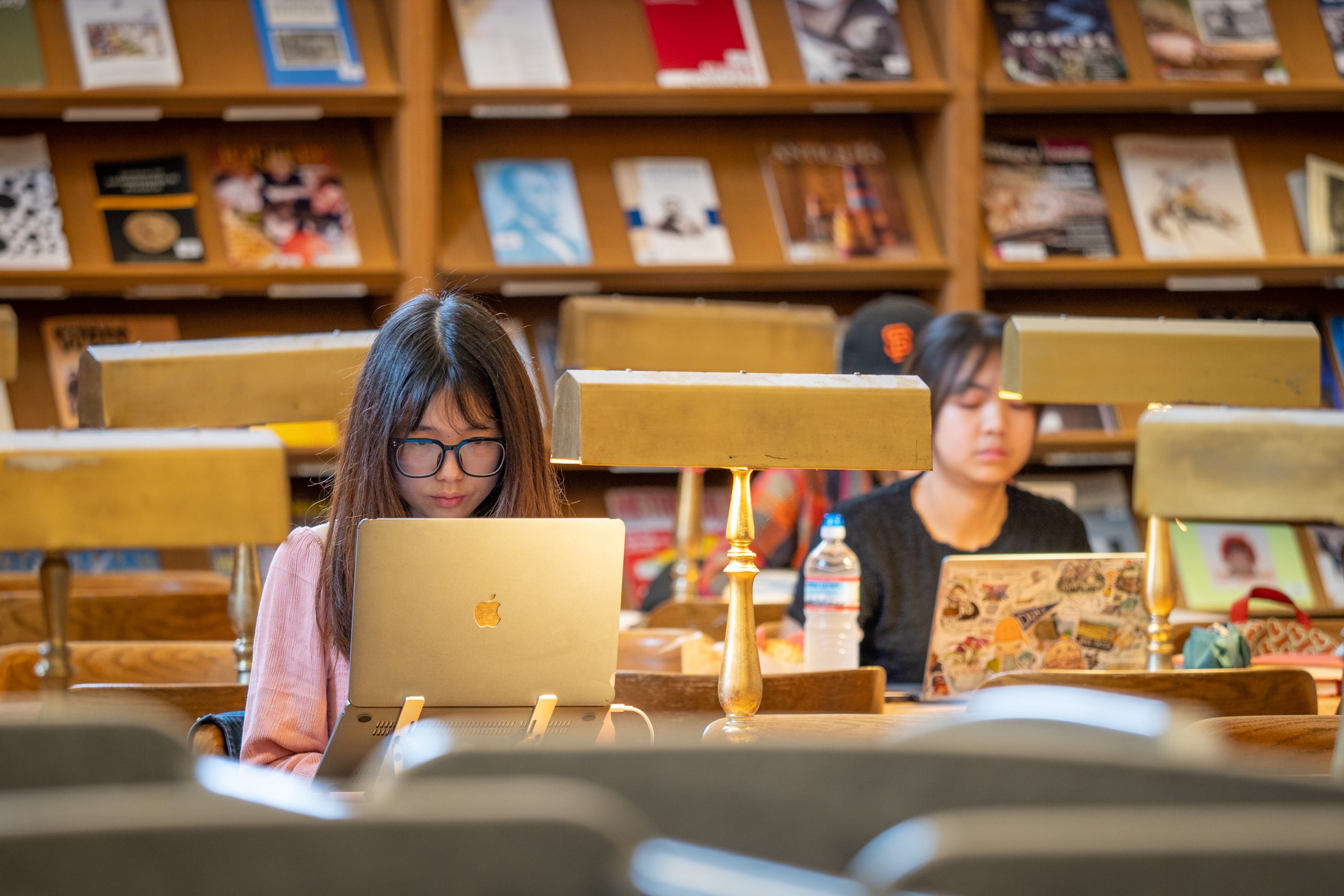The image captures a scene inside a library, viewed from the perspective of someone seated. The focus is on two young Asian women engrossed in their work on laptops amidst a studious atmosphere. 

The woman on the left, wearing black-rimmed glasses and a pink shirt, has long, straight brown hair parted in the middle. She is intently looking at her MacBook, which is mounted on a stand, allowing a clear view of its iconic silver Apple logo. 

To the right and slightly behind her sits another woman clad in a black shirt, with black hair pulled back. Her laptop is adorned with a multitude of stickers, including a prominent blue Duke pennant flag. In front of her is a squirt-type water bottle. 

Behind the woman with the sticker-covered laptop, a man in a plaid shirt and a baseball cap can be discerned. 

The background of the library features three rows of slanted bookshelves stocked with magazines. Each desk in the library is equipped with distinctive lamp fixtures—golden rods extending straight up, capped with horizontal mailbox-shaped lights. At the bottom of the image, slightly blurred, there appears to be the tops of grey chairs.